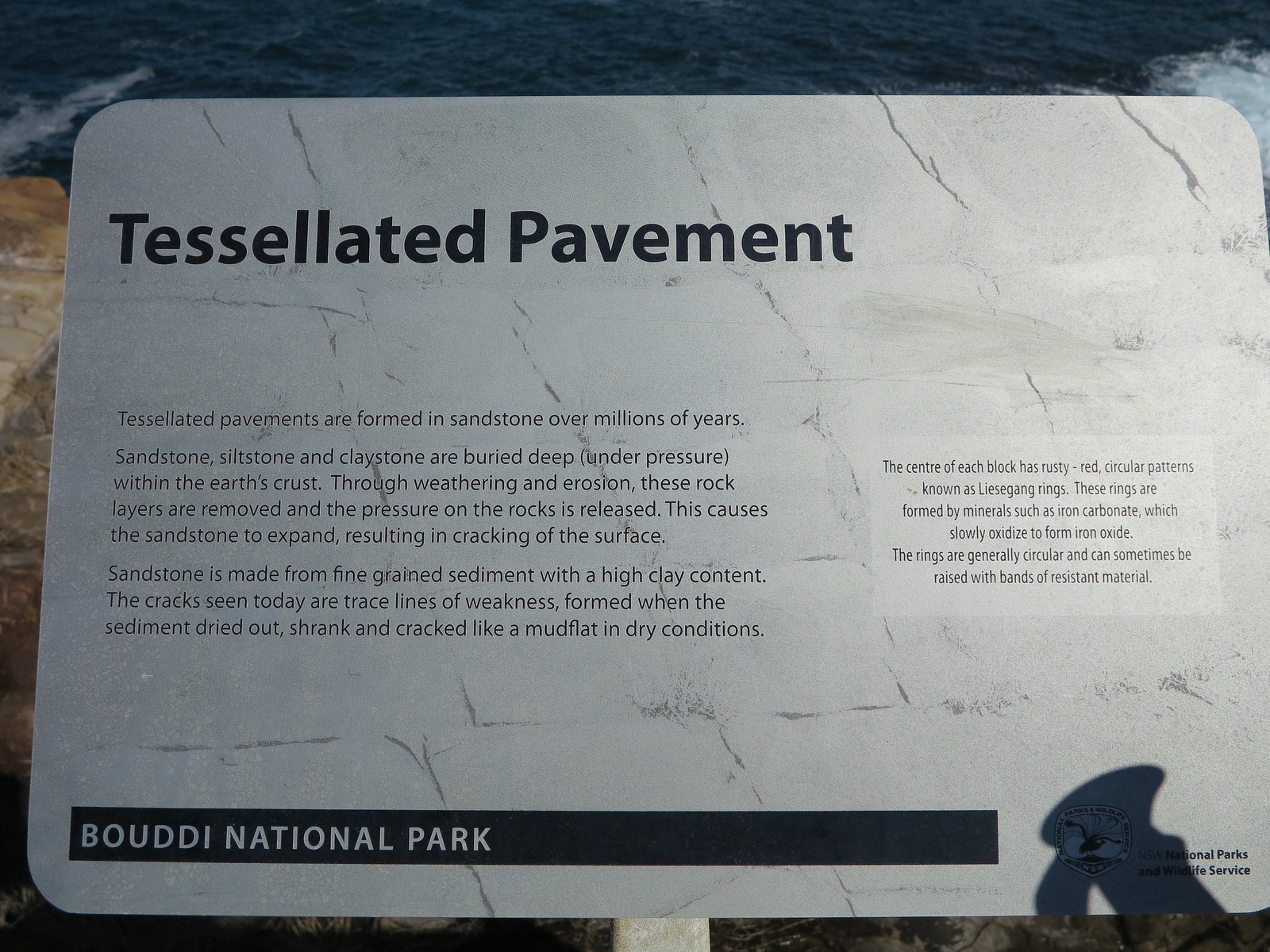This photograph captures a white, rectangular plaque with rounded edges, prominently featuring the heading "Tessellated Pavement" in black letters at the top left corner. The plaque, set against a scenic backdrop of a blue ocean and brown stones, explains the geological formation of tessellated pavements, detailing the millions of years of sandstone, siltstone, and claystone compression and subsequent expansion that create distinctive surface cracks. The sign, mounted on a white pole visible at the bottom center, dominates the image and includes several sections of black text, including a faint gray rectangle filled with additional detailed descriptions. At the bottom of the plaque, a horizontal black strip bears the inscription "Bouddi National Park" in white, along with an indistinguishable symbol and text partially obscured by a shadow. The setting appears to be the edge of a rocky cliff, suggesting an outdoor, mid-day scene with natural tones of blue, brown, tan, off-white, black, white, and gray.